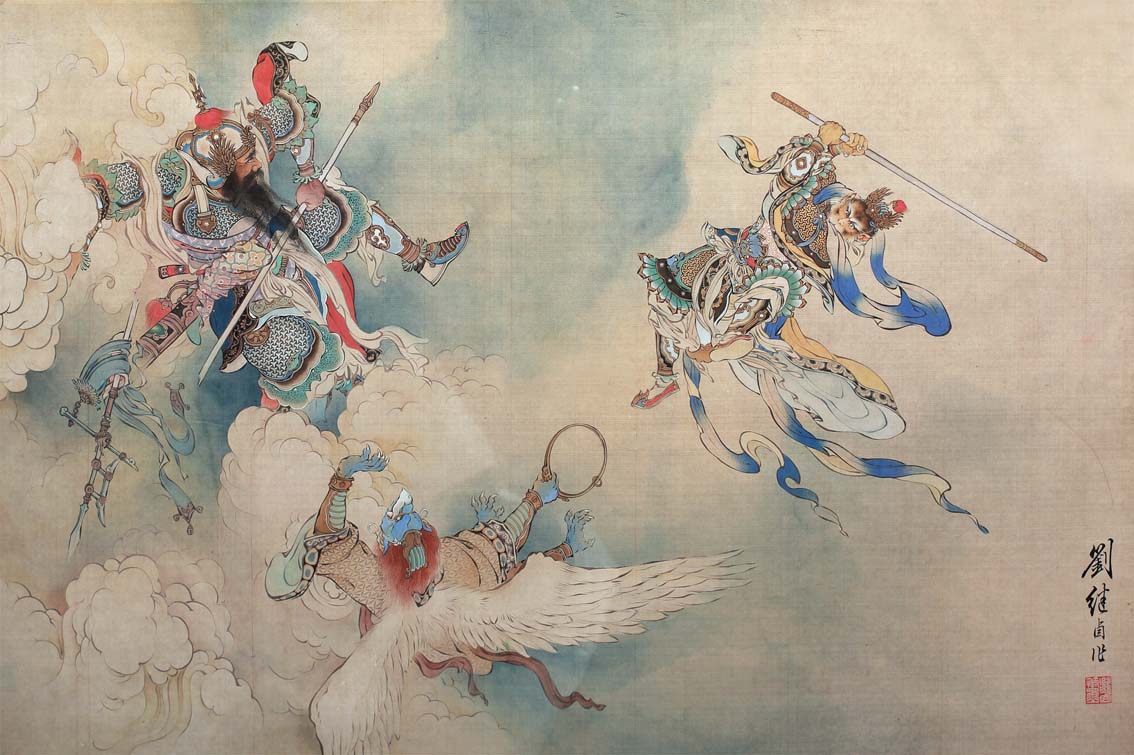This intricate painting illustrates a captivating fantasy scene set amidst the clouds, featuring three Asian figures resembling samurais or angels. The bottom right corner of the artwork is adorned with Asian characters, likely Japanese or Chinese. On the far left, a warrior with a long black beard clad in ornate, multicolored armor and a decorated headpiece wields a staff. On the bottom left, another ethereal figure has wings and holds a golden ring, dressed in flowing cloth that resembles a poncho. The figure on the upper right also grasps a staff, donning unique blue and green robes with armor. The detailed depiction of these airborne swordsmen or samurai warriors presents an enchanting and serene celestial narrative.